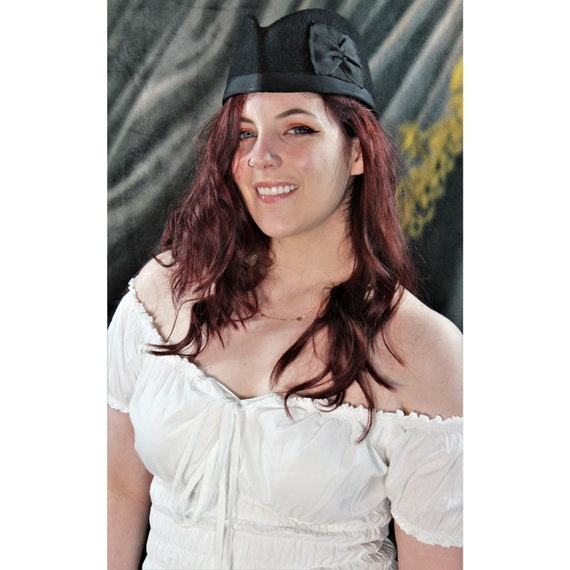In the photograph, there is a young woman in her early to mid-20s with striking dark auburn hair. She has a pale complexion complemented by her choice of light makeup, including copper or bronze eye shadow and stylistic black eyeliner, giving her a captivating cat-eye look. Her dark eyebrows frame her eyes nicely, adding to her expressive appearance. A delicate gold necklace adorns her neck, and she sports a nose piercing in her right nostril. 

She is dressed in an off-the-shoulder white peasant top with a ruched and form-fitting design that ties above the breasts and cinches around the waist, somewhat evoking traditional Bavarian attire. 

Her head is crowned with a distinctive black fedora-like hat, embellished with a bow on top and satin edging, which adds a touch of elegance to her look. She stands against a background of black curtains adorned with yellow embellishments or lace. The woman smiles warmly, her straight white teeth accentuating her radiant demeanor, as she looks directly at the camera.